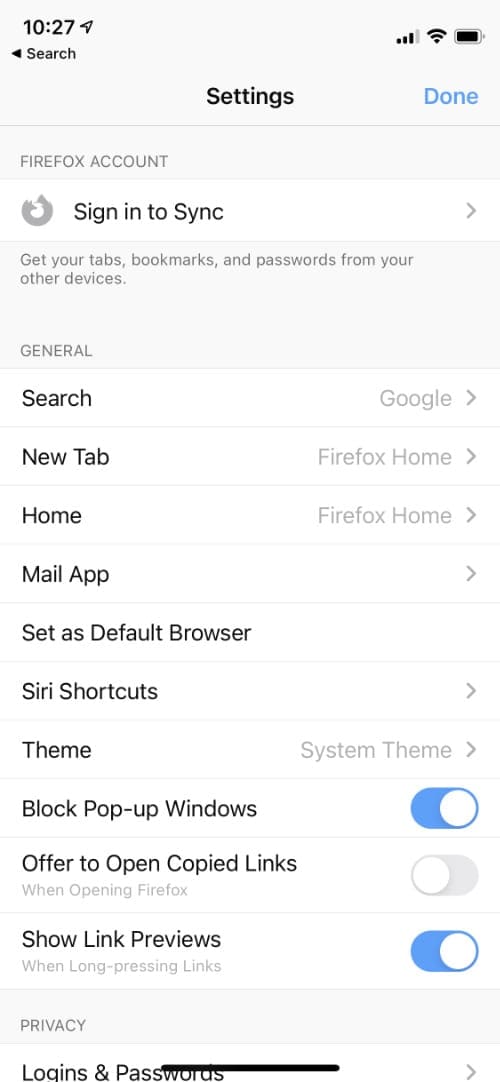This is a detailed screenshot from a mobile phone. At the very top, in the left corner, there is a small gray rectangle displaying the time "10:27" in black font. Next to it, there is a location-sharing icon. To the right, there are icons representing the Wi-Fi signal, mobile signal strength, and battery status.

Beneath this top bar, in large black font, the word "Settings" is prominently displayed. Next to it, to the right, the word "Done" is written in blue font.

Below, a gray rectangle contains the text "Firefox account" in a darker gray font. Following that, a white rectangle features a logo of a refresh arrow with the text "Sign in to sync." This is followed by a smaller gray font that reads, "Get your tabs, bookmarks, and passwords from your other devices."

Further down, the menu items listed include various options: 

- "General"
- "Search"
- "Google"
- "New tab"
- "Firefox Home"
- "Home"
- "Mail app"
- "Set as default browser"
- "Theme" with a subtext of "System theme"
- "Siri shortcuts"
- "Theme"

The layout and design elements suggest that this screenshot is from a settings menu within the Firefox browser app on a mobile device.